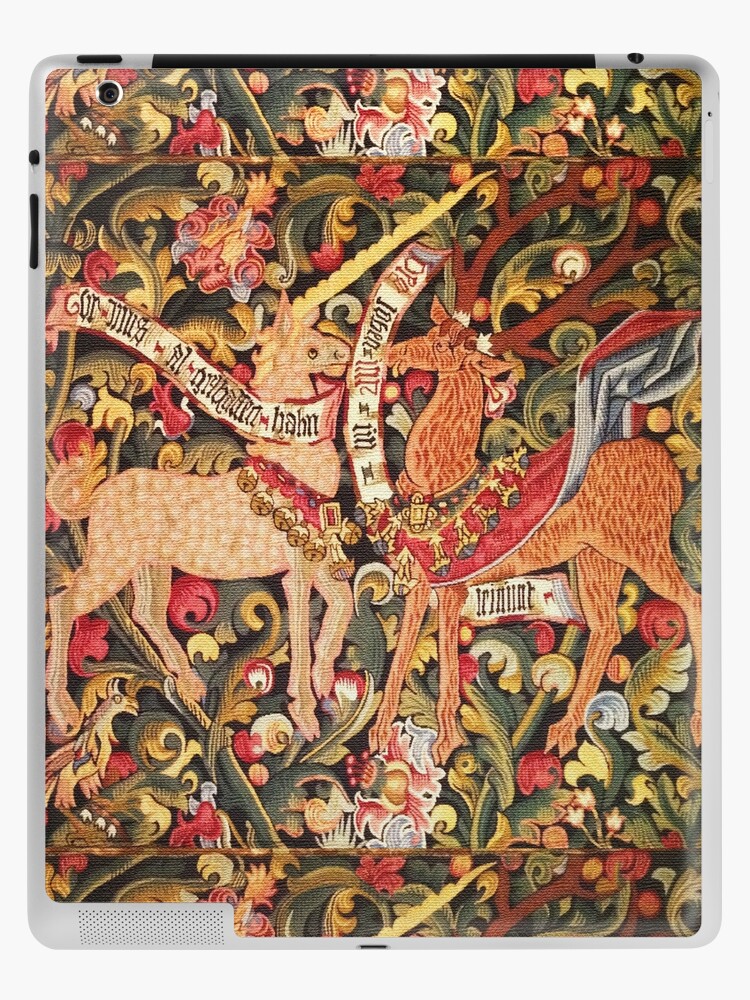This product listing image showcases a detailed iPad or tablet cover, set against a pristine white background that emphasizes its intricate design—a high-quality close-up ideal for online shopping. The cover, likely suited for an Apple iPad, features a vibrant and elaborate backdrop filled with green and golden-yellow floral patterns and curly leaves. At the center of the cover, two majestic animals, resembling deer with hooves, stand facing each other. The one on the left is a light tan with white spots and adorned with a red collar featuring golden bells and a white banner around its neck. The deer on the right, darker brown in color, wears a red cape with golden jewels hanging from its neck. Both animals are framed by an abstract, floral tapestry-like design that adds an old-world charm to the modern accessory. Despite the unreadable text in a foreign language on the banners, the cover's artistic depiction and attention to detail make it a captivating choice for enhancing the aesthetics of a tablet.